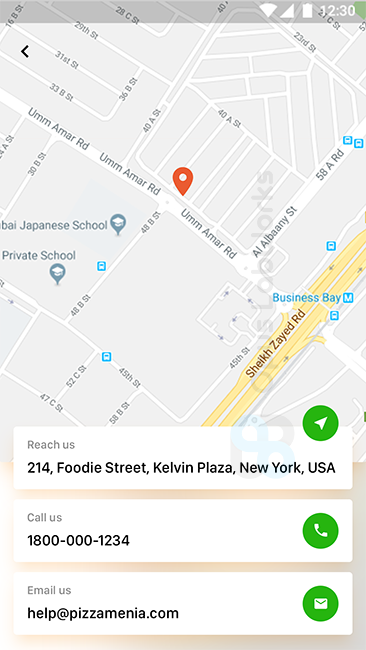In the image, a smartphone displays Google Maps in portrait orientation, roughly twice as tall as it is wide. The top of the screen features a transparent gray status bar containing several white icons: a fully filled Wi-Fi signal icon, a full cellular connection indicator, a fully charged battery symbol, and the time displayed as 12:30. 

Dominating the screen is the Google Maps interface. At the center of the map, a prominent red pinpoint marks a specific search location. The map showcases various towns and street names that are difficult to pronounce. Notable landmarks include "Business Bay" highlighted in blue, several bus stops, a partial listing for a Japanese school, and a private school.

Towards the bottom of the screen, there are three white, landscape-oriented rectangular boxes. The first box is a "Reach Us" section displaying an address: "214 Foodie Street, Kelvin Plaza, New York, USA," accompanied by a navigation arrow. The second box is a "Call Us" option featuring a green phone icon. The third and final box is an "Email Us" option showing the email address "help@pizzamania.com," with a green email icon, inviting users to reach out for assistance.